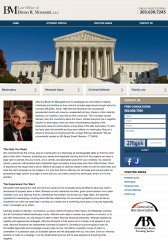The image depicts a website dedicated to a professional man, most likely a lawyer. At the center of the page is a prominent photograph of the man, who is dressed in a suit and positioned in front of a bookcase, suggesting a scholarly or legal setting. Although much of the text and numbers on the webpage are blurry, the website's focus is clear. In the upper right-hand corner, a phone number is visible, enabling visitors to contact the individual or the firm.

A large, detailed image of a grand, stone-pillared building, possibly a courthouse or capitol, dominates another section of the webpage. This building features eight imposing pillars at its entrance, reinforcing the legal theme. Upon closer examination, the words "Law Office" and the initials "BM" are faintly discernible within the textual content of the page, further confirming the legal nature of the site.

Overall, the website appears to belong to a law firm, with the photographed man being a key attorney or representative of the practice. The architectural imagery of the stone building underscores the firm's connection to the legal profession.